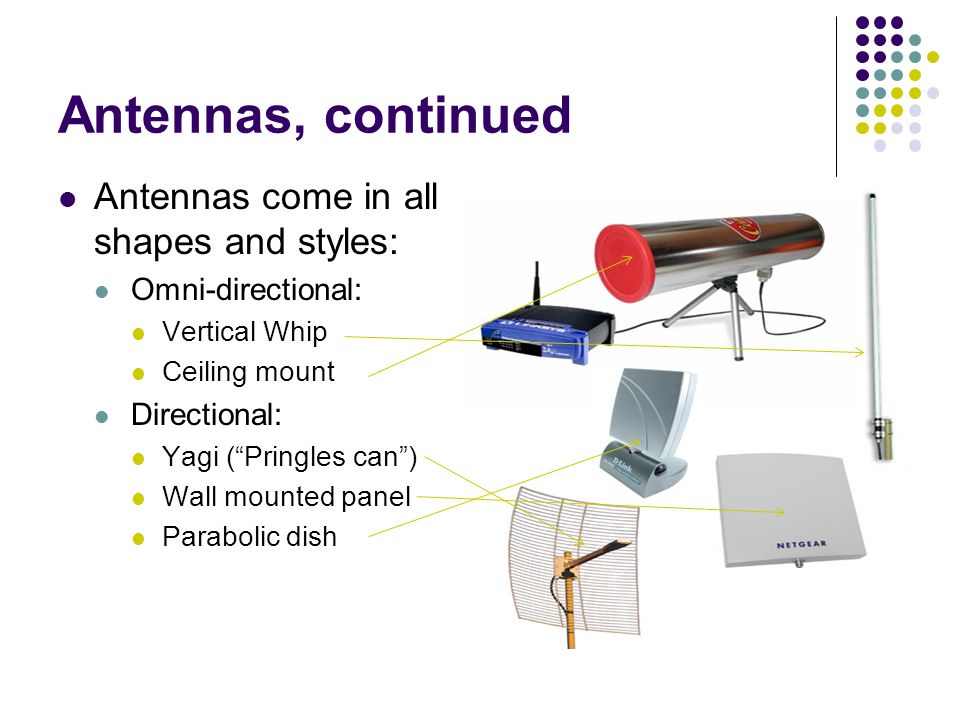The image showcases a series of various antennas, each with distinct shapes and designs, positioned on the right side, while the left side contains descriptive information and a corporate logo in the upper corner. The antennas depicted include:

1. A silver, canister-shaped antenna with a prominent red end.
2. To its left, a black, straight antenna resembling one typically connected to a modem.
3. A silver, upright square antenna resting on a foldable platform.
4. Below that, a traditional roof antenna with a rounded square panel featuring lines and a pointing element.
5. A grey, square, wall-mounted panel antenna with a coax cable outlet.
6. Further right, a thin, rod-like antenna.

The text on the left explains that antennas come in all shapes and styles, emphasizing two main categories: 
- **Omni-directional antennas**, including vertical whip and ceiling mount types, with lines pointing to the can-shaped and long rod antennas.
- **Directional antennas**, such as Yagi (compared to a Pringles can) for the roof antenna, wall-mounted panels for the grey square one, and parabolic dishes for the silver folding platform.

Additionally, the antennas are identified by their manufacturers, including Netgear and D-Link.